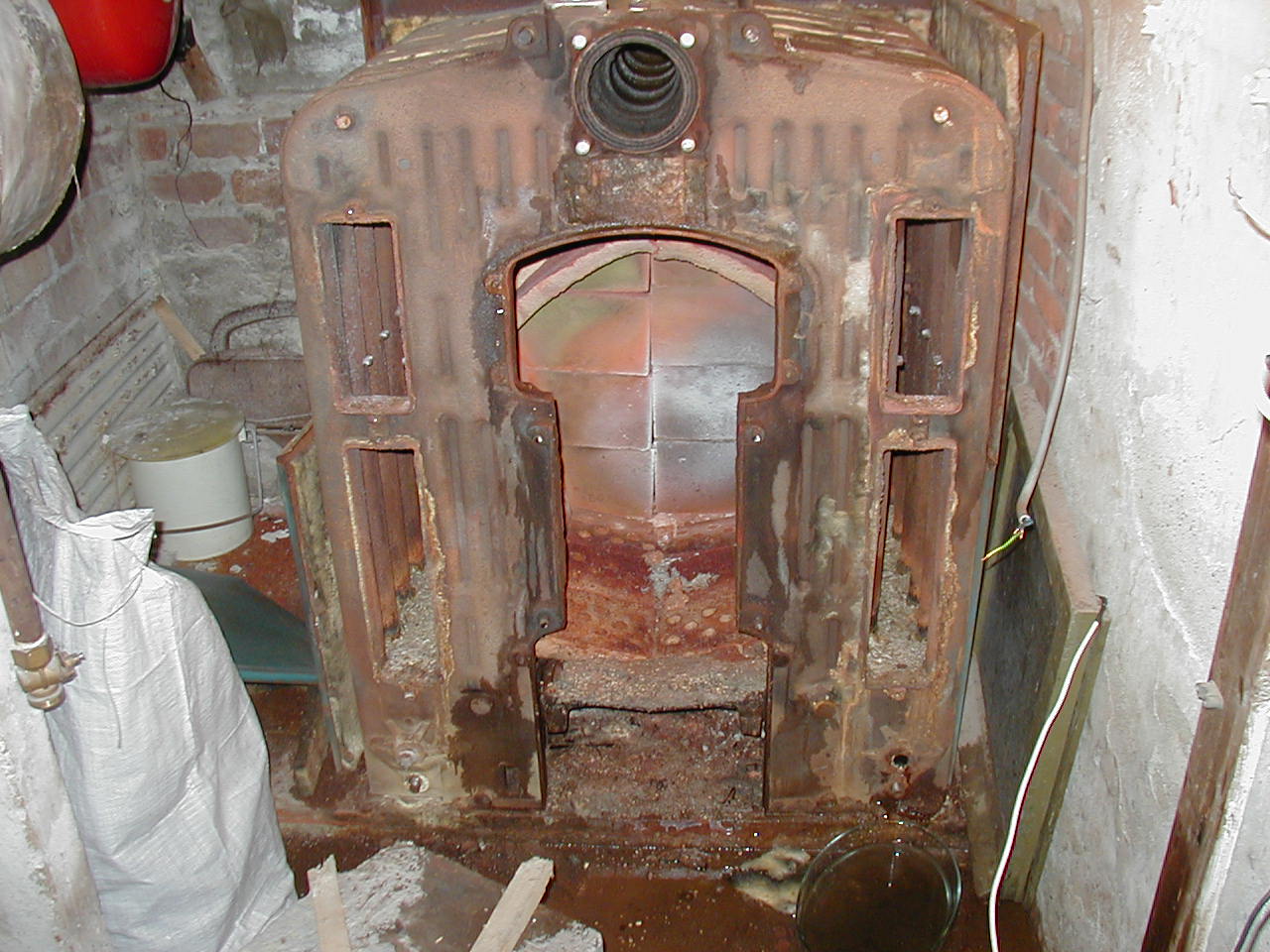In a small, dank, and possibly basement room with a mix of painted and exposed brick walls, there stands an ancient, metallic, and rusty piece of equipment. This device, reminiscent of a radiator or boiler unit, is positioned near the left-hand side of the image. The device is brown, possibly a furnace or some sort of ancient boiler, and features a round hole at the top, likely intended for a hose, with vents on its upper corners. A rubber gasket with a tube is visible, along with a rectangular section of plaster with curved edges and four vertically-aligned rectangles on either side. Various objects are scattered around—towards the bottom left, a white tarp partially covers something next to a can of paint, and nearby, there's a blue ledge and a bowl of dirty water at the bottom right. Above, objects hang from the wall, including a gray item and a red one, and there are wires protruding from the device. The overall condition of the room and the equipment suggests it has not been in operation for a long time.